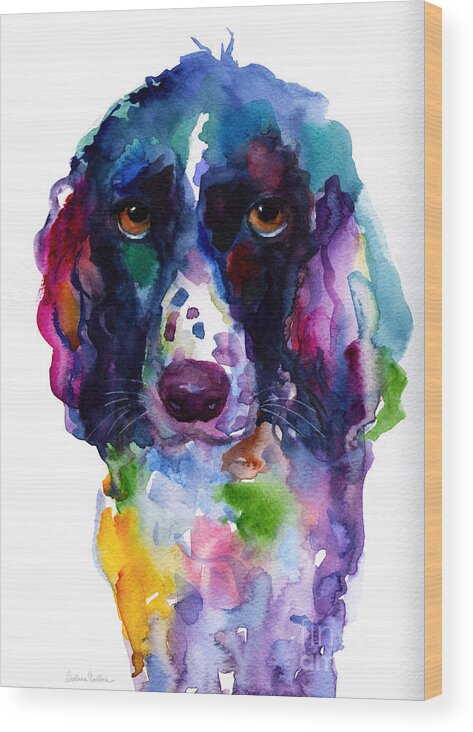The image is a brightly lit, high-clarity photograph of a watercolor painting on a white canvas. The painting prominently features a dog adorned with a vivid array of colors that deviate from its natural hues. The dog is positioned centrally within the frame, with a particularly detailed focus on its face, which includes white fur surrounding a dark purple nose and brown eyes. The dog's head is framed by long, somewhat shaggy hair. The left ear is dark with pink highlights, while the right ear showcases blue and purple accents. The dog's body, illustrated in an abstract style, incorporates colors such as purplish hues on the right, yellow on the left, blue outlining the belly, and a mix of pink and green within the belly area. The canvas itself is angled slightly to the left, revealing its thickness, which is bordered by a light brown or gray tape along the right edge. A small, illegible signature appears at the bottom left corner of the canvas.